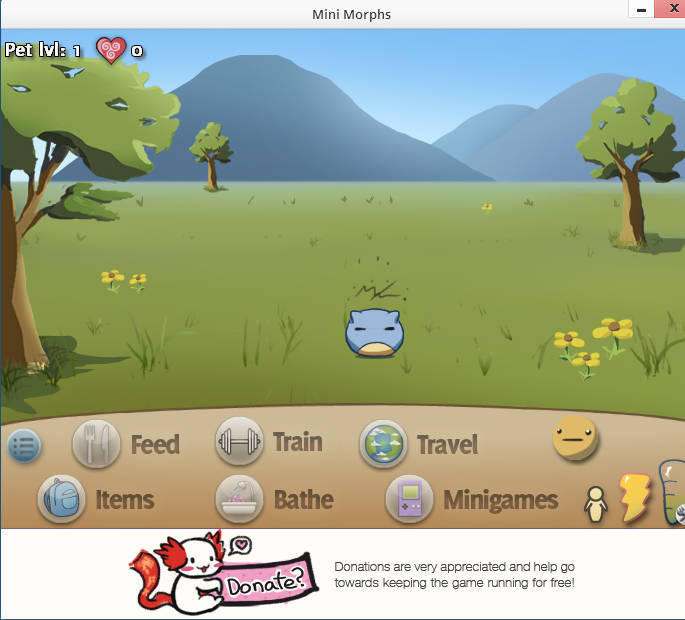This image appears to be a screenshot from a digital pet simulation game, either on a computer or a phone. At the very top, it features a gray border typical of a window interface, complete with various control buttons including a red 'X' button for closing the window on the right side. 

Dominating the center of the screen is a vibrant scene. The background showcases a clear blue sky stretching across the frame, with two sets of gray mountains flanking either side—one on the left and one on the right. Below the mountains is a spacious area of lush green grass. Three trees are strategically placed within the scene: one in the bottom left, another in the upper middle left, and the third on the far right.

In the upper right corner of the image, text reads "Pet Level 1" alongside an icon of a heart with a zero next to it, indicating the pet's current status or affection level. The focal point on the grass is a small blue creature with a white belly and simple line-drawn eyes.

Near this creature, yellow flowers resembling daisies add a splash of color to the greenery. Below the main scene, a brown menu area provides various options for interacting with the pet: “Feed,” “Items,” “Train,” “Bathe,” “Travel,” and “Minigames.” Also present is a circle icon, likely a mood indicator, showing two dots for eyes and a straight line for a mouth, accompanied by a lightning bolt symbol which could denote energy or activity.

At the very bottom of the screen, there is a "Donate" button featuring an illustration of a fantastical creature with a tail and flaming red ears, emitting a heart from its mouth, possibly encouraging in-game support or contributions to the developers.